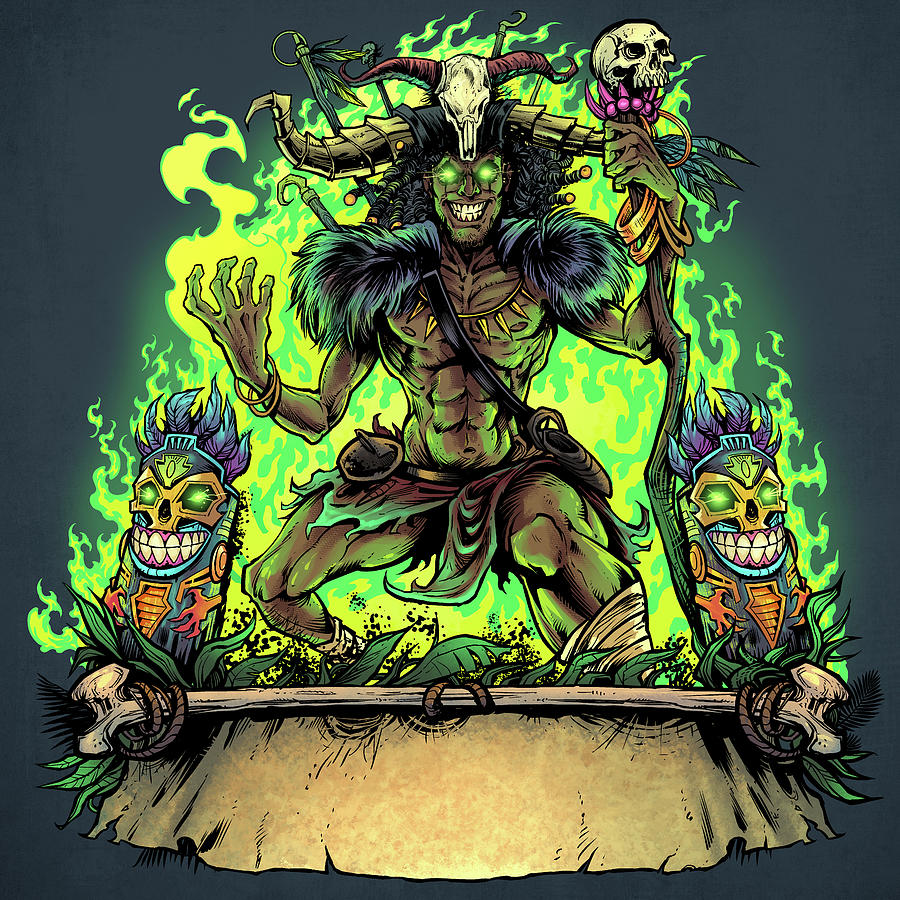The image is an animated drawing depicting a muscular, dark-skinned man with a mystical aura. Centered in the image, the man is adorned with various tribal elements: an imposing animal skull headdress with horns, and a striking spiky yellow necklace. His attire is minimal, consisting of a torn leather wrap around his waist and an animal fur draped over his shoulders. 

He holds a wooden staff topped with a white skull that lacks a lower jaw, resting amidst a pink flower-like crown, accompanied by gold bangles on his wrists and the staff. His eyes glow a vibrant green, echoing the large, green flame with a white center that surrounds him, creating an ethereal backdrop. 

The flanking figures resemble tiki or Easter Island statues with gold skeleton faces, large white teeth, and glowing green eyes. These twin statues have red claw-like hands positioned on their midsections and wear elaborate headdresses with purple feathers tipped in blue.

The scene is set against a dark green background, with the man standing on a wooden base covered in grass. A large animal bone with ropes and a draped cloth stretches across the bottom of the image, hinting at a ritualistic or ceremonial context. The overall setting is bright and detailed, bringing to life the mystical and tribal essence of the scene.